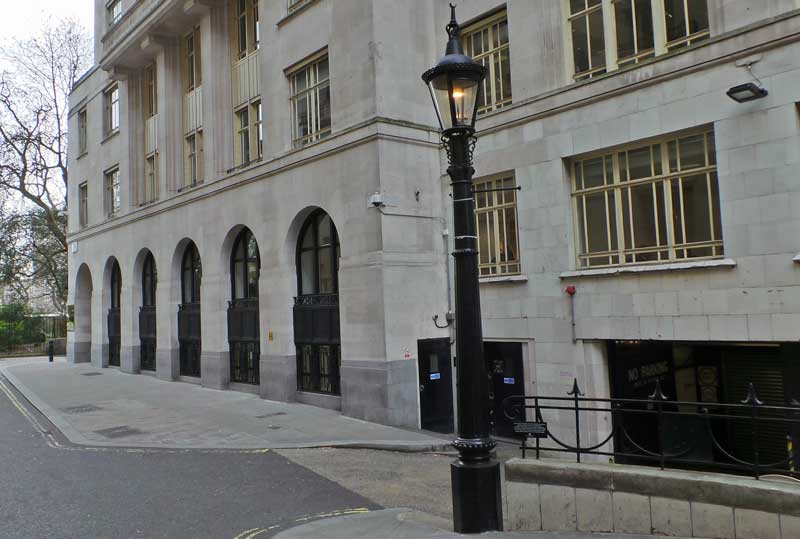This detailed photograph captures a multi-story, tan cement building in a landscape orientation. The entire backdrop showcases this four-story structure, characterized by its light brown beige stone walls and an orderly arrangement of six brown arches on the main floor, centered toward the left. Each arch exhibits wooden interiors with four window panes visible on each side, and a distinctive glass arch at the bottom.

A broad cement sidewalk stretches across the entire foreground, leading directly to a classic black lamppost that stands prominently at the bottom center, extending to the top center of the photo. This old-fashioned lamppost is minimally adorned with occasional white strips, culminating in a glowing orange-yellow light at its apex.

Adding to the architectural charm, the building features an underground parking driveway, hinting at a functional urban setting. The bottom right section of the image shows darker windows and a cast iron fence, along with a "No Parking" sign on a door, reinforcing the urban landscape feel.

Notable as well, the second floor showcases yellow-paned windows, further adding to the building's old-world character, reminiscent of structures found in historical parts of the UK, Paris, or London. The top left corner of the image captures the subtle outlines of trees, completing this picturesque urban scene.